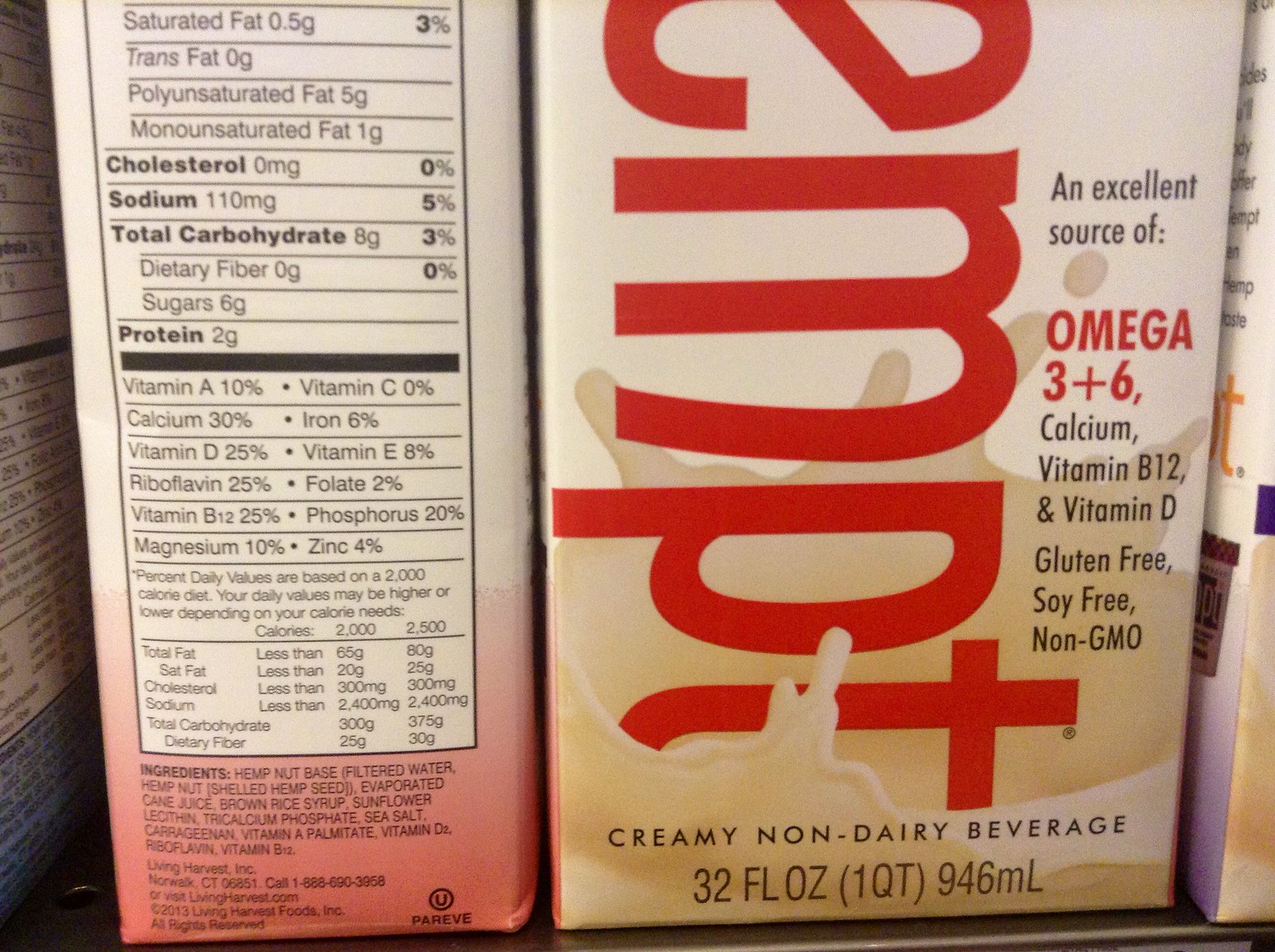A rectangular container of a creamy non-dairy beverage is prominently displayed. The container is predominantly white with light brown accents, creating a visually appealing contrast. Large, bold red letters showcase the product's name, although part of the label is cut off, adding a touch of mystery. The side of the container proudly advertises its nutritional benefits, highlighting it as an excellent source of Omega 3 and 6, calcium, vitamin B12, and vitamin D. Additionally, the beverage is marketed as gluten-free, soy-free, and non-GMO, catering to a variety of dietary needs. At the bottom of the container, the quantity is clearly marked as 32 fluid ounces. Beside the main container, another similar carton is positioned on its side, revealing the actual list of ingredients and detailed nutritional information for the product.